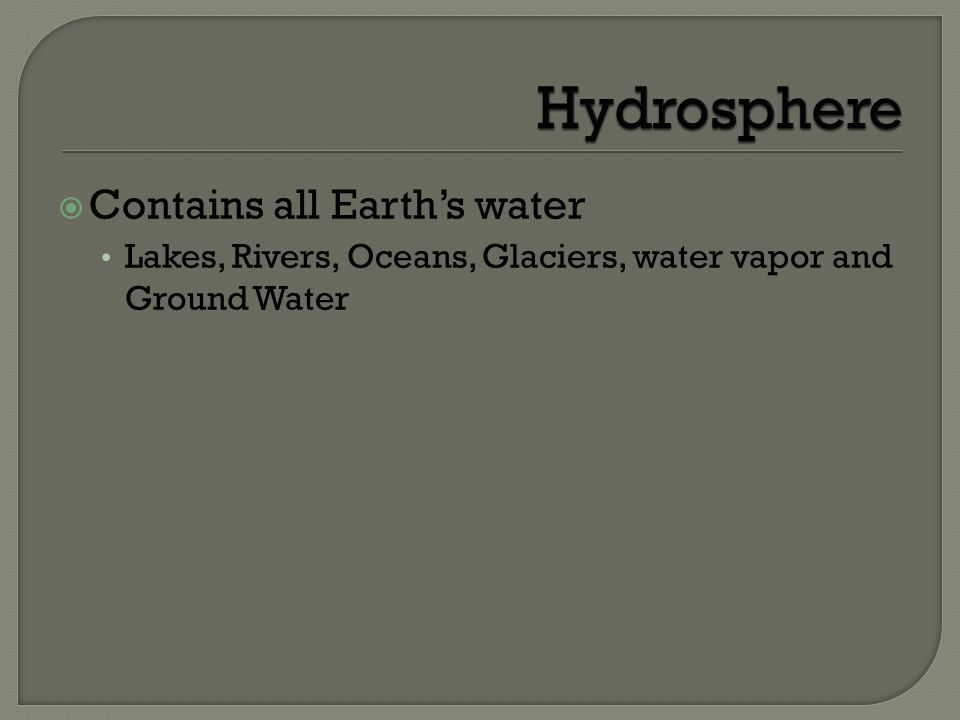The image, likely from a slide in a presentation, features a title "Hydrosphere" in bold, black text positioned in the upper right-hand corner. The background is a dark, olive green color, and the title is emphasized by an underlying green horizontal line. The slide includes a main bullet point, marked by a green dot, stating "Contains all Earth's water." Indented beneath this is a sub-bullet point in white that lists "lakes, rivers, oceans, glaciers, water vapor, and groundwater," all in black text. The text maintains proper capitalization except for "water vapor." Surrounding the slide is a lighter olive-colored frame with rounded corners at the top left and bottom right, contrasting sharply with the slide's otherwise squared-off edges. The detailed layout, color scheme, and textual elements suggest an informative and visually coherent design.